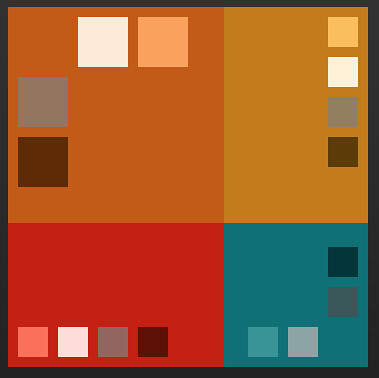The image features a large dark gray square divided into four smaller, equal-sized quadrants, each with distinctive color themes and smaller squares within them. The top left quadrant is an orange-brown shade, showcasing four smaller squares in light brown, white, gray, and dark brown. The top right quadrant has a deeper butterscotch brown background, with four smaller squares arranged vertically in light brown, white, gray, and dark brown. The bottom left quadrant is red, containing four smaller squares in dark red, gray, white, and light orange. Finally, the bottom right quadrant is a teal color, with its smaller squares organized in a unique pattern: gray and light gray running vertically, and teal and light gray situated horizontally. The entire image is bordered with a dark brown or black trim, giving it a clean, framed appearance.